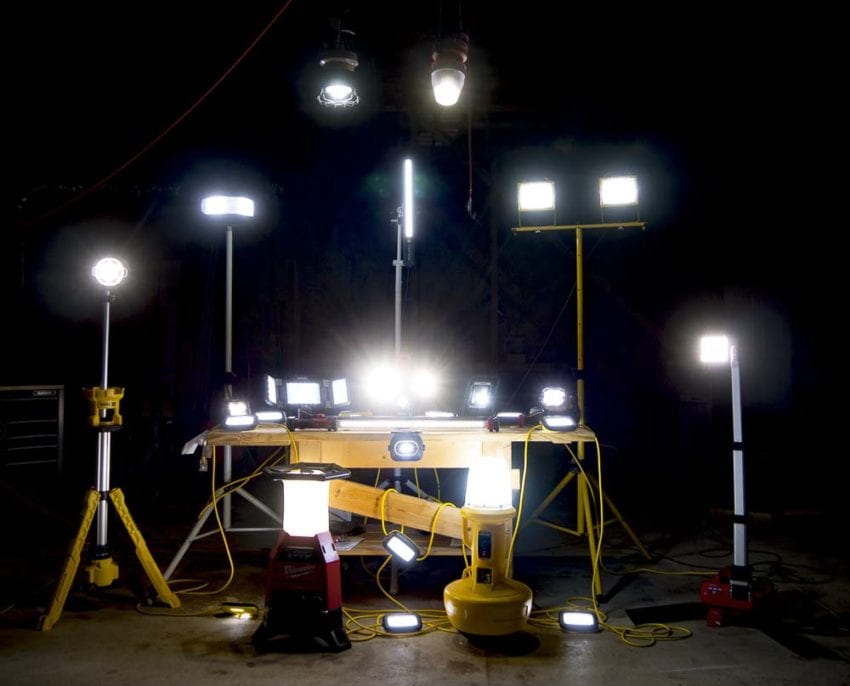The image showcases a variety of work lamps arranged in a visually striking formation against a black backdrop. There are five main standing lamps at differing heights, all facing the viewer. At the center, the tallest lamps dominate the scene: a dual-round light on a tripod and a rectangular bar light slightly higher next to it. Hanging from the central tripod are two lights, one round and one cylindrical. Adjacent to these, there is another tripod featuring two connected rectangular lights, and a final silver tripod hosts a solitary rectangle light at a lower height.

In front of these standing lights is a yellow table, adorned with four more work lamps, primarily square in shape with the brightest, roundest one positioned at the center. The table contrasts against the dark background and seems to have a drawer with a black symbol on it, hinting at its potentially metallic composition. On the ground, two additional cylindrical work lamps provide a splash of color, with a red lamp on the left and a yellow lamp on the right. The entire setup suggests a detailed lighting demonstration, akin to what might be used for a worksite or a film set, emphasizing the diversity and functionality of the lighting equipment on display.